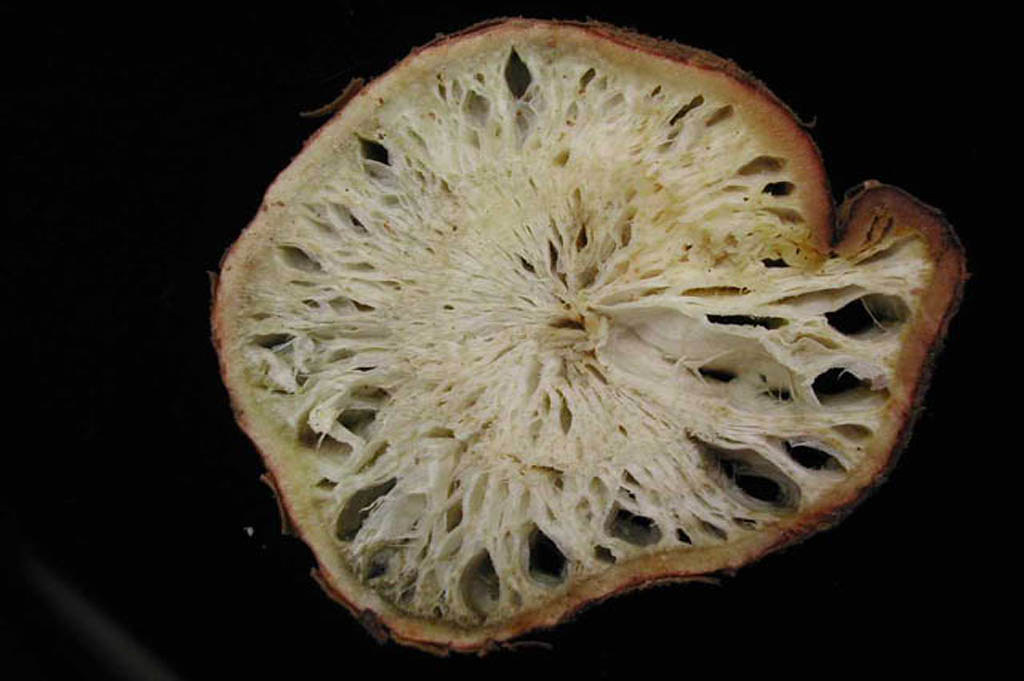This image is a close-up, detailed view of a round, porous object set against a pitch-black background. The object appears to be a dried slice of fruit or possibly a loofah. It has a dark brown edge that looks like a crust or rind. The interior is mostly white with a hint of yellowing in some areas. The white center is filled with numerous airy, dark holes, giving it a porous texture. The level of detail suggests the image might be taken under a microscope, capturing fine intricacies such as folds and internal structure. There is no text on the image, and the predominant colors are black, brown, and white.